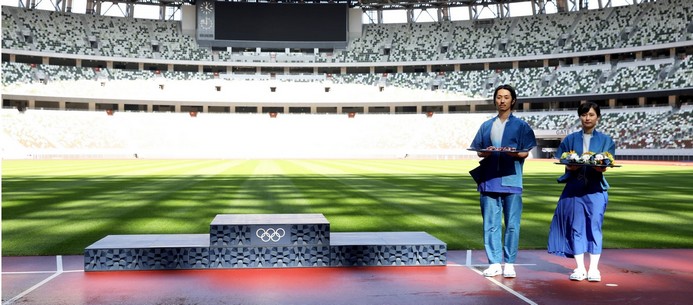In a sunlit stadium, an image captures a delayed award ceremony for an Olympic event. The background reveals an expansive auditorium with vacant seat tiers and a prominent, switched-off display screen on the upper level, framed by clock designs and possible glass windows. The sun's rays illuminate a lush green field behind two people on a brown patch of ground with white markings. Prominently in the foreground stands a three-tiered Olympic podium, the iconic Olympic logo adorning the highest tier. To the right of the podium, a man and a woman, both with black hair and dressed in blue traditional attire with white shirts, jackets, and shoes, stand poised. The man holds a platter, likely bearing medals, while the woman’s tray seemingly carries flowers, ready to honor the victorious athletes.